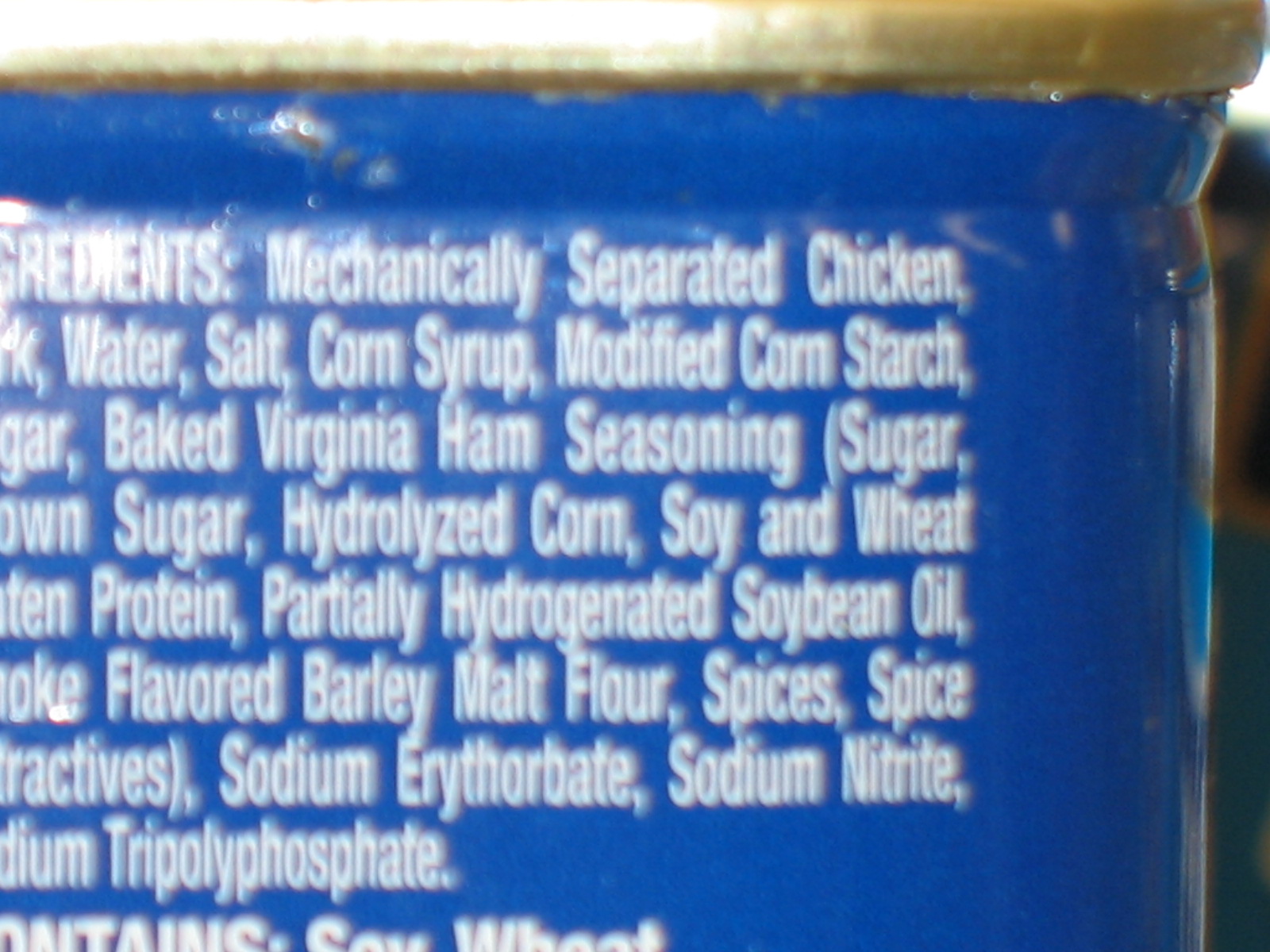This detailed photograph captures a close-up view of the right side of a blue can, showcasing its ingredients list. The image reveals the golden or brass rim adorning the top of the can, adding a touch of elegance. The left edge of the can is not visible, with the text slightly cut off. The word "Ingredients" appears at the top of the list, although the letter "G" is partially missing. The ingredients are listed in a white font against the blue background. Towards the bottom of the list, the word "Contains" is visible but partially cut off, displaying only from the mid-section of the letter "O" to the right. Next to it, the allergens "soy" and "wheat" are clearly listed.